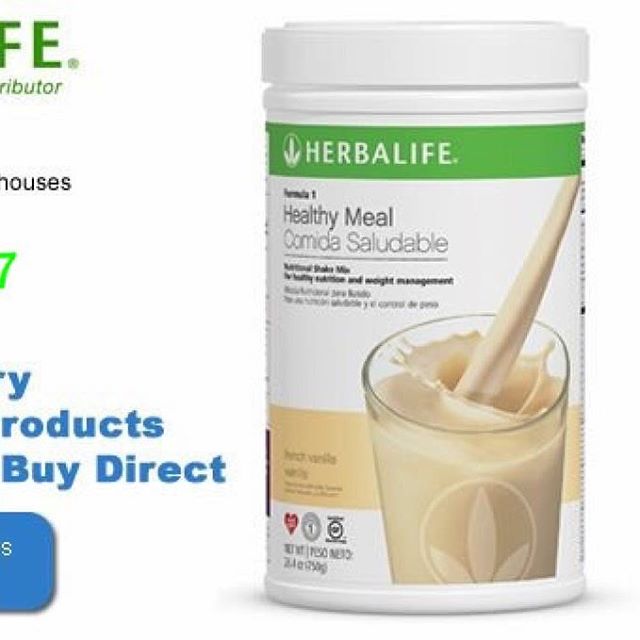The image appears to be a screenshot from a website featuring a product advertisement for a meal replacement shake made by Herbalife. The background of the image is entirely white. The focal point is a white plastic canister with a white cover cap. The canister features a green and white label. Prominently displayed on the label is a large glass filled with what looks like beige-colored milk. The label reads "Healthy Meal" prominently, and below that, the same phrase is written in Spanish. In the bottom left corner of the label, "vanilla" is indicated, suggesting the flavor of the shake. The Herbalife logo, composed of the words "Herbalife" in white on the green band and accompanied by a symbol of three white leaves in a circle, is also clearly visible on the label. The wording on the right-hand side is mostly cut off and blurred, making it difficult to read.